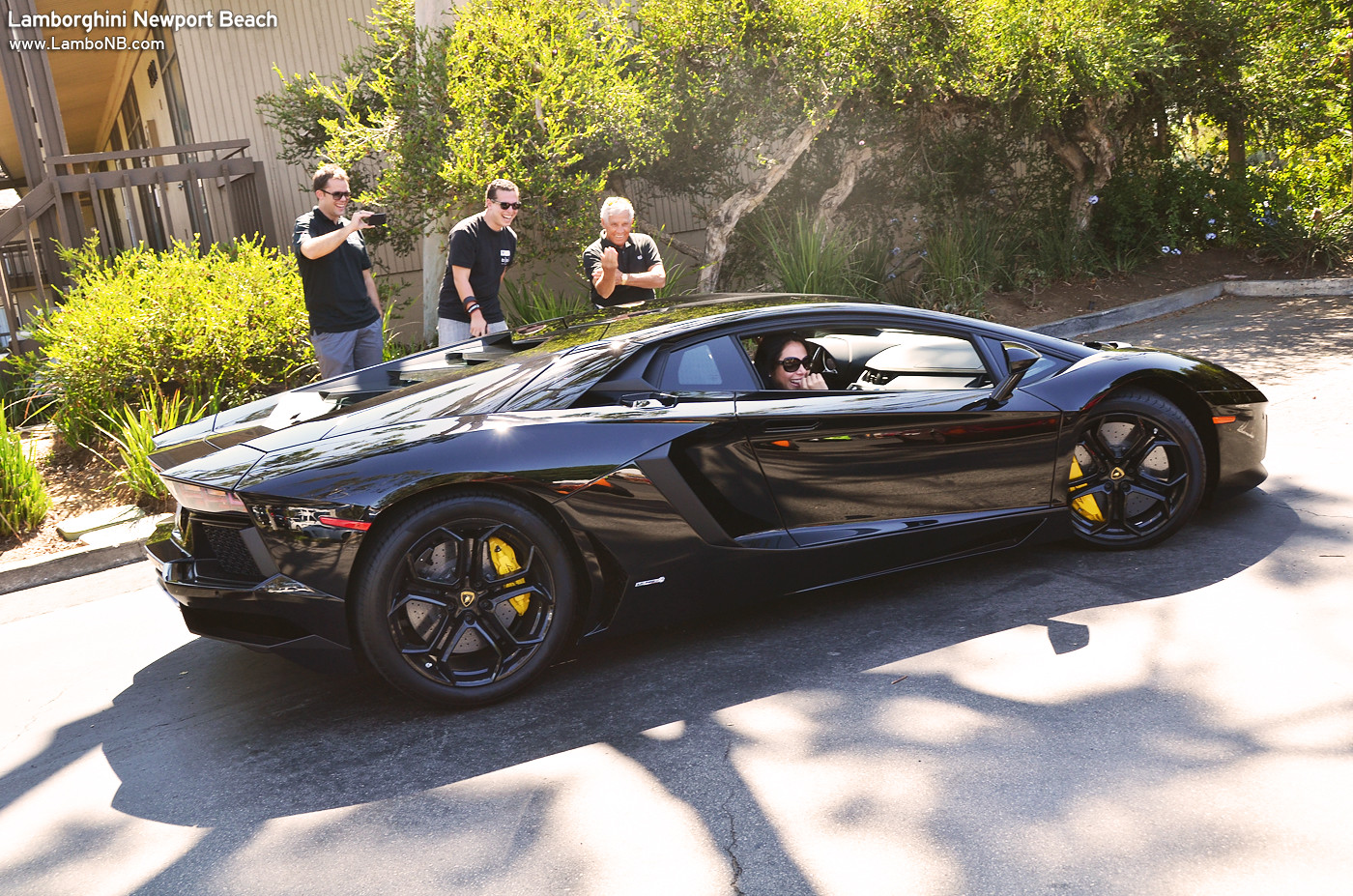The image features a sleek black Lamborghini positioned in the middle of a sunny asphalt street, facing to the right. Sunlight streams down, casting the car's shadow sharply against the pavement. In the passenger seat, a woman with black hair and wearing black sunglasses smiles warmly out the open window, adding a touch of human connection to the scene. Surrounding the vehicle on the driver's side are three men, all clad in black t-shirts and distinctively accessorized with sunglasses. The man on the far left holds a smartphone horizontally, seemingly capturing the striking car in a picture or video. The middle figure, with noticeable hairbands on his right wrist, shares in the group's relaxed, laughing camaraderie. The oldest of the trio, with gray hair, stands to the far right, engaging in the shared moment with something in his hand. The backdrop features verdant trees and cultivated bushes, and a stone wall that gives structure to the scene. At the upper left, a building bears the signage "Lamborghini Newport Beach," hinting at the high-end locale, with a web address displayed beneath the bold print.